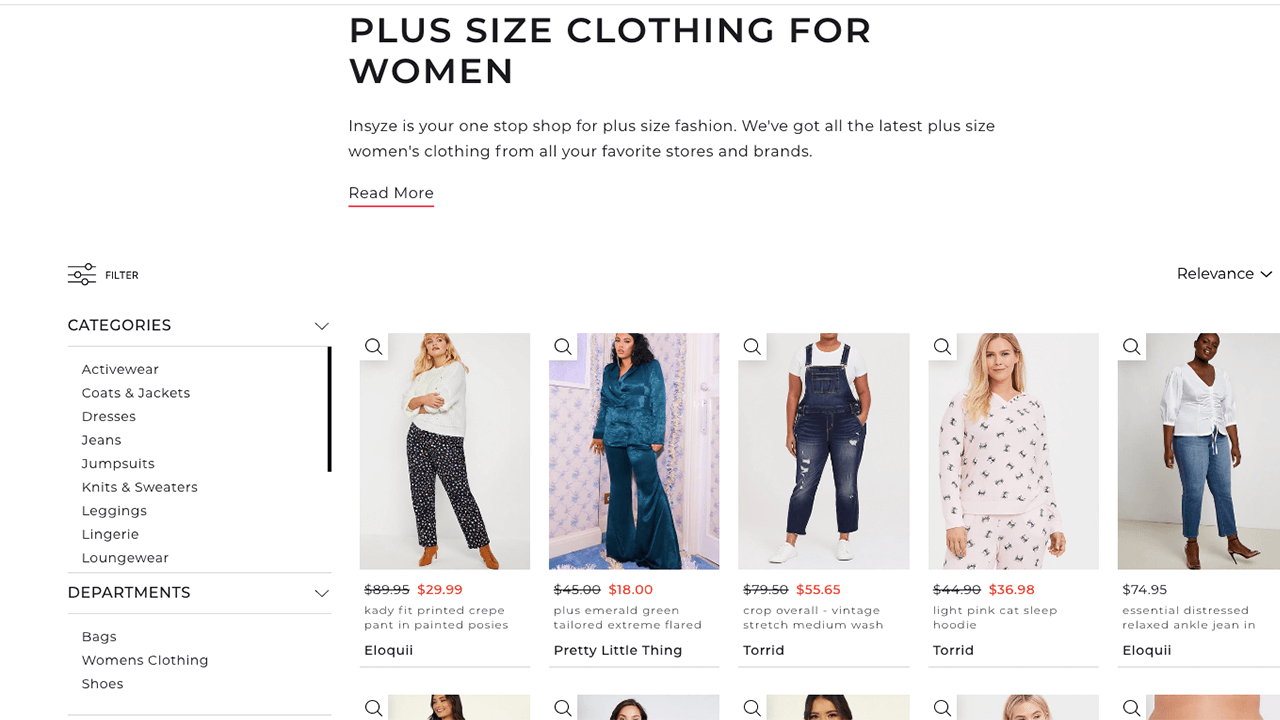Screenshot of an online shopping website for plus-size women's clothing. 

At the top center, there is a banner that reads "Plus-Size Clothing for Women" in large, bold text. Below it, there's a brief paragraph with "read more" underlined in red in smaller letters, indicating additional information is available.

The background of the page is entirely white, providing a clean and uncluttered look. On the left side of the screen, there's a vertical navigation menu listing various clothing categories: Active Wear, Coats & Jackets, Dresses, Jeans, Jumpsuits, Knits & Sweaters, Leggings, Lingerie, and Loungewear. Below these categories, there are additional department options displayed with a collapsible caret, including Bags, Women's Clothing, and Shoes. A scrollbar on the right side of this menu indicates that more categories can be browsed by scrolling.

The main section of the page showcases images of models wearing different outfits arranged in a grid. There are five images visible in the top row:
1. The first model is wearing cozy pajamas.
2. The second model is in satin pajamas.
3. The third model sports jean overalls.
4. The fourth model appears in another set of comfortable pajamas.
5. The fifth model wears jeans paired with a chic top.

Above these images, in the top-right corner of the main section, there's a sorting option labeled "Relevance" with a caret indicating it can be expanded for other sorting methods. 

Just below the visible row of images, a second row starts, showing the tops of the models' heads, hinting at additional outfits that can be revealed by scrolling down.